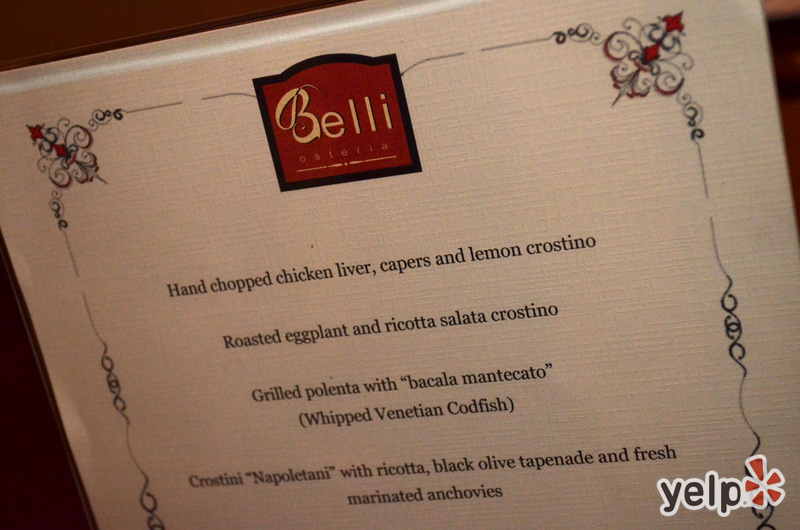This photograph features a close-up of a slightly slanted restaurant menu against a burgundy background, with the lower right corner displaying the "Yelp" logo accompanied by a five-cornered clover symbol in brown and white. The menu page itself is light pink with a decorative border featuring symbols in the top corners. At the center top of the menu, the restaurant's logo reads "Belli" in white or yellow lettering on a brown background, with "Astoria" written in a smaller font beneath it. Below the logo, the menu lists several items: "Hand-chopped chicken liver, capers and lemon crostino," "Roasted eggplant and ricotta salata crostino," "Grilled polenta with bacala mantecato, whipped Venetian codfish," and "Crostini Napoletani with ricotta, black olive tapenade, and fresh marinated anchovies."